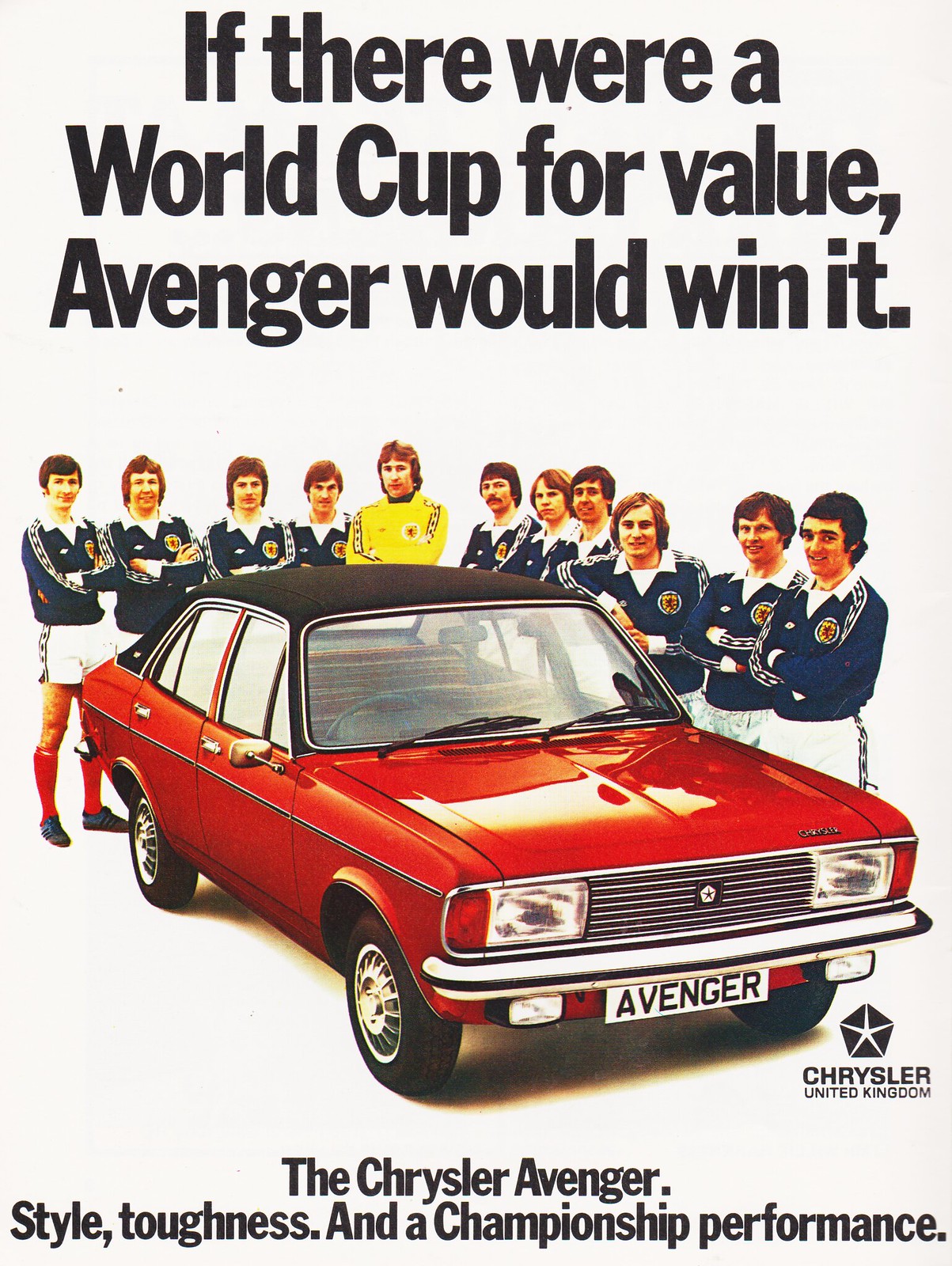This detailed vintage advertisement features a red Chrysler Avenger with a convertible black top and white wheels, prominently showcased in the center. The car's license plate reads "Avenger." Surrounding the car is a football team of 11 individuals, 10 players and one coach. The players are wearing blue shirts and white shorts, while the coach, positioned centrally, is distinguished by a yellow shirt. Above the image, in bold black text on a white background, the headline reads: "If there were a World Cup for value, Avenger would win it." Below the car, the advertisement continues with the tagline, "The Chrysler Avenger – style, toughness, and a championship performance." The overall design and attire of the people suggest a retro look from the 1970s or 1980s, likely aimed at a UK audience, as indicated by the inclusion of "Chrysler United Kingdom" within the ad. The team members are depicted with their arms folded, leaning on the car, and smiling, further emphasizing the Avenger's appeal and association with championship performance.